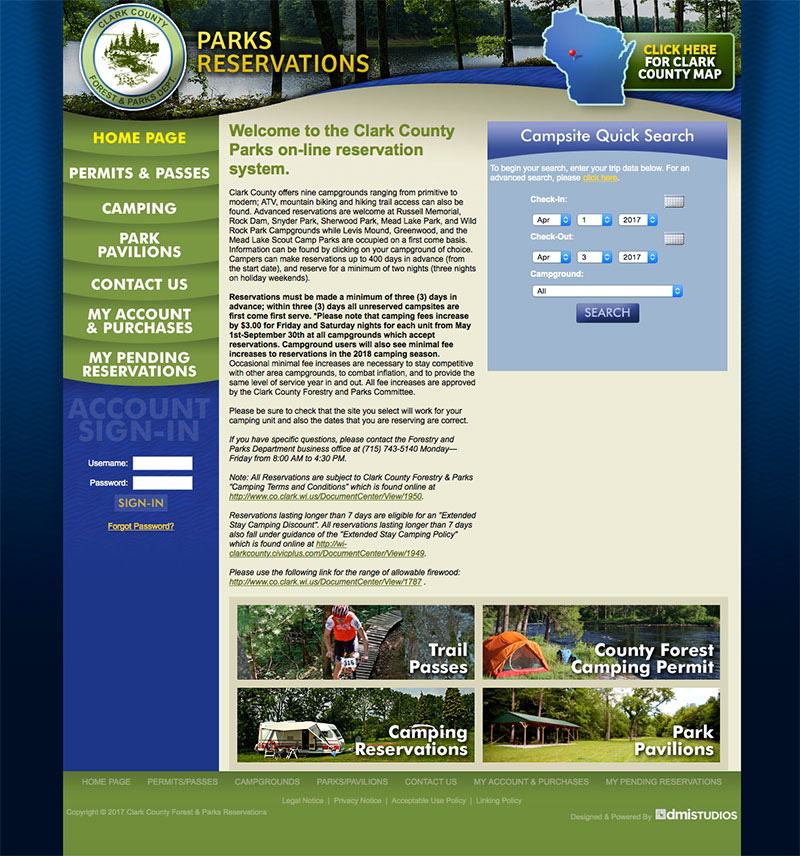**Caption:**
A screenshot captures an older-style Clark County Forest and Parks Department website, featuring a detailed layout and navigation system. The site is framed by gradients transitioning from blue to dark blue or black on either side. At the top is a wavy banner housing a circular crest on the left, featuring green tree illustrations on a white background with the text "Clark County Forest and Parks Department." Adjacent to this, yellow text reads "Parks" and "Reservations" beneath it. To the right of the banner, there’s a map of Wisconsin with a pinpoint, accompanied by a green box with yellow text stating "Click Here" and white text reading "for Clark County Map."

On the left sidebar, sections are highlighted in green with yellow text indicating selections. The first highlighted section, "Homepage," is followed by white text links: "Permits and Passes," "Camping," "Park Pavilions," "Contact Us," "My Account and Purchases," and "My Pending Reservations." Further below, a blue section prompts users to "Account Sign-In," featuring fields for username and password, a sign-in button, and a "Forgot Password" link.

The main content area sports a light yellow background with green text welcoming users to the Clark County Parks Online Reservation System, though the detailed text is unreadable. On the right side, a blue box with a dark blue banner is titled "Campsite Quick Search," likely equipped with functionality to search campsite availability, culminating in a search button at the bottom.

At the bottom of this section are four images, each paired with captions in white text highlighting different park services: "Trail Passes" next to a cyclist, "County Forest Camping Permit" beside a tent by a lake, "Camping Reservations" with an RV, and "Park Pavilion" featuring a cabin. Finally, a green banner at the bottom, presumably containing site navigation links, rounds out the page, though its text is not fully discernible.